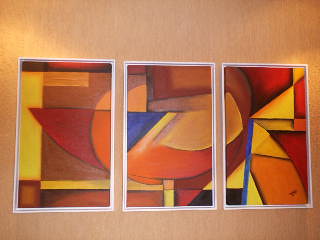This photograph captures a striking work of art composed of three vertical rectangular panels, each encased in thin white frames and mounted against a light brown background tinged with a peach hue. Illuminated by a golden light from both sides, the panels collectively form a cohesive abstract composition reminiscent of early 20th-century Cubism. The artworks feature a vivid interplay of geometric shapes rendered in a palette of red, orange, yellow, blue, and dark brown. Notably, the left panel includes a shape resembling the end of a knife, while the middle panel evokes the stem and bowl of a wine glass. A small black patch is conspicuously located at the bottom of the middle and right panels, adding a dramatic contrast. The overall effect is one of dynamic patterns and interlocking shapes that do not represent any particular objects but rather emphasize the harmony and tension between the forms and colors.